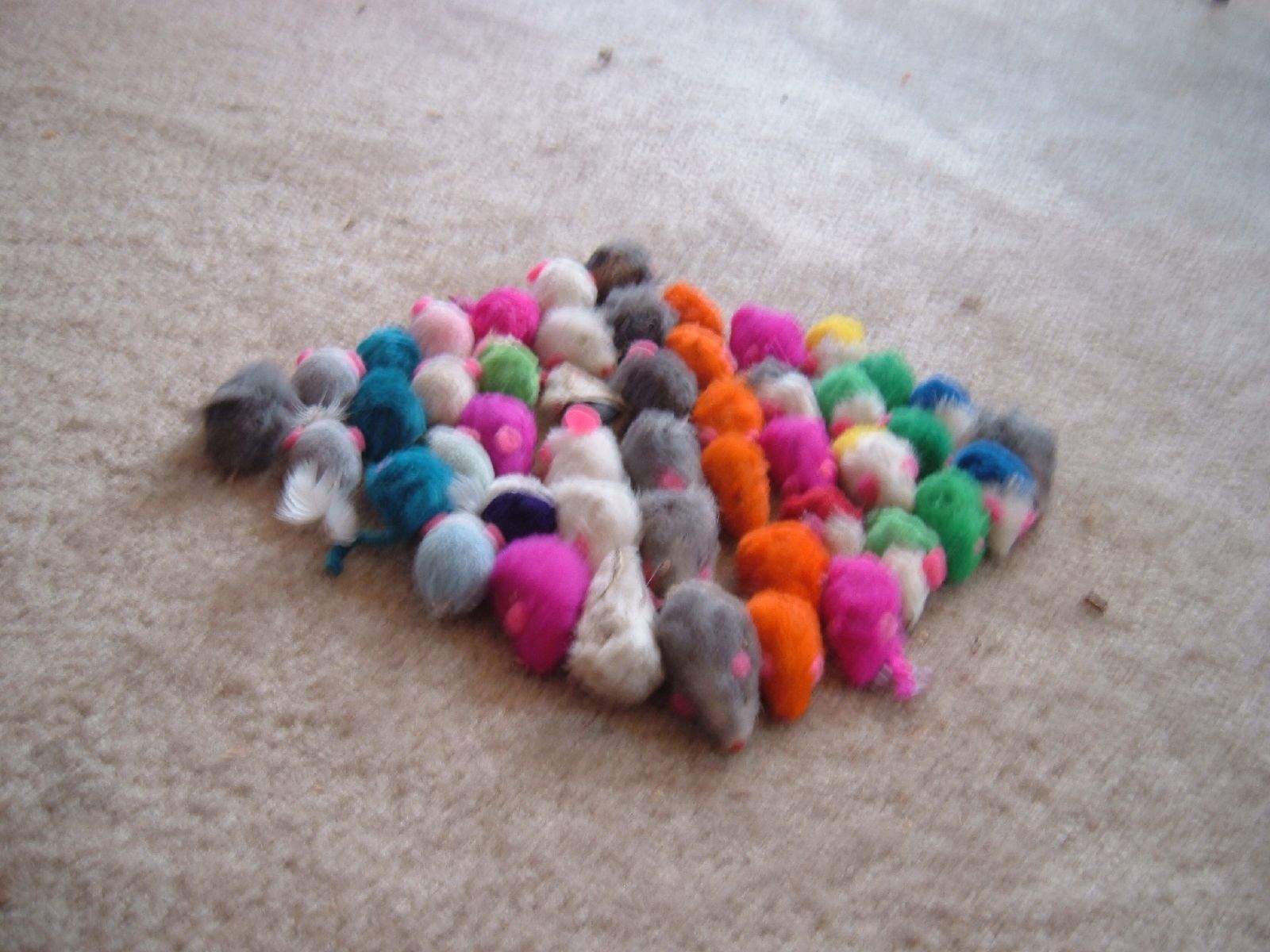The image features a symmetrical, diamond-shaped arrangement of pet toys resembling mice, displayed on a short, cream-colored shag carpet that is noticeably dirty and covered with debris. Despite the blur, the toys are identifiable by their mouse-like shape and size, characterized by gray bodies with pink ear-like areas. Centered perfectly are six gray mice forming a vertical line from tip to tip of the diamond. Flanking the gray row on the right are successive rows of orange, pink, mixed colors containing green, three green, two blue, and a lone gray toy. On the left side are rows of white, predominantly pink, off-white, three blue, two gray, and another single gray. The toys are meticulously lined up by color, creating a striking, star-like pattern, with slight variations in color placement adding to the intricate design.